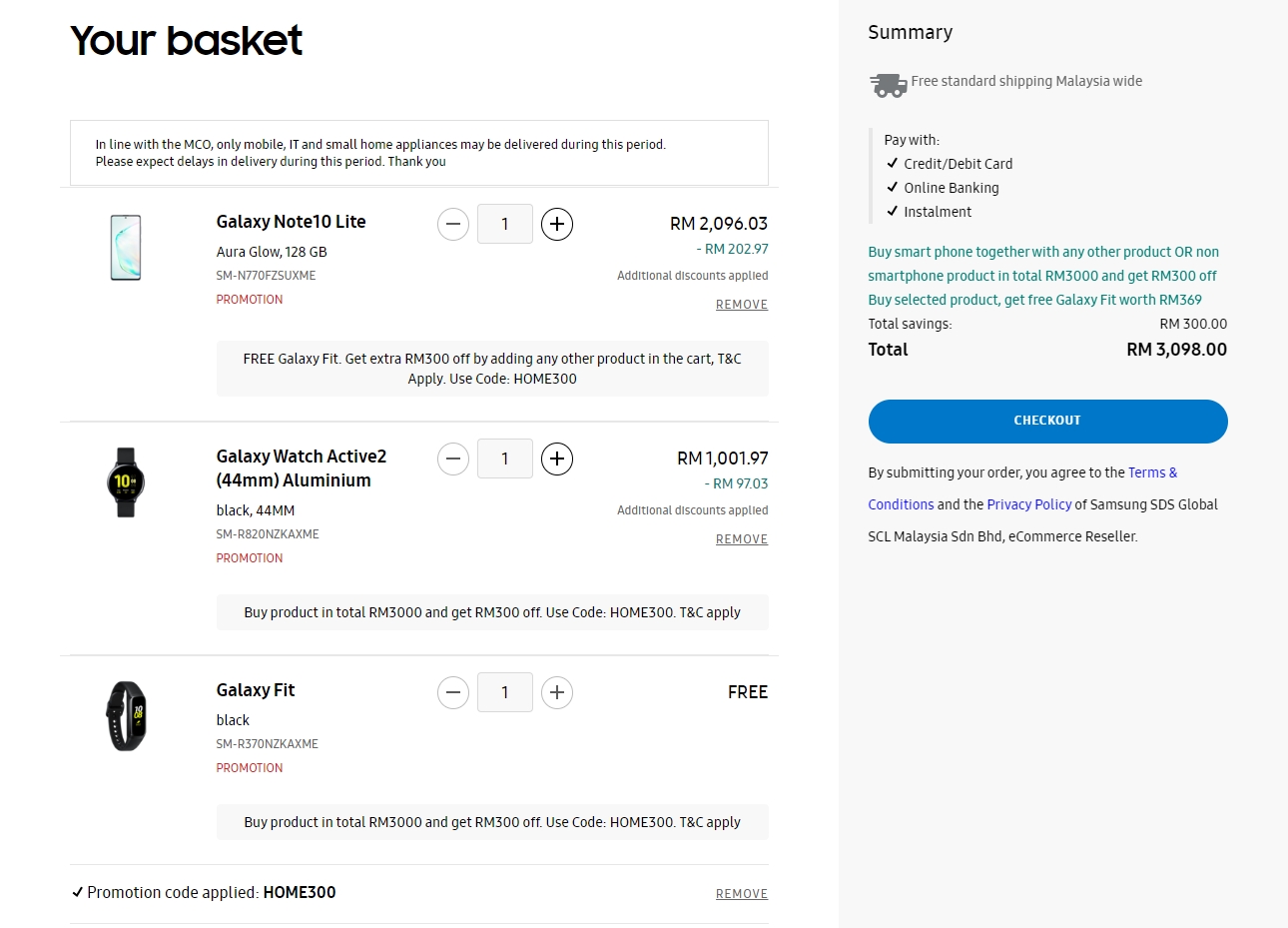The image depicts an online shopping interface detailing the user's current shopping cart and promotions available. On the right side, a prominent dark black bold heading reads "Your Basket". Below, a notification informs customers that only mobile IT and small home appliances may be delivered during this period, with an advisory to expect delays in delivery. 

Highlighted in red is a promotion for a Galaxy Note 10 Lite (Aurora Glow, 128GB, model SM-N770FZSU). The item has been added to the cart at a price of RM2,096.03. Additionally, a free Galaxy Fit is included with the purchase. An extra discount of RM300 can be obtained by adding another product to the cart using the code "Home300," subject to terms and conditions.

Further down, another product, the Galaxy Watch Active 2 (45mm, Aluminum), is displayed, which has also been added to the cart, priced at RM1,001.97.